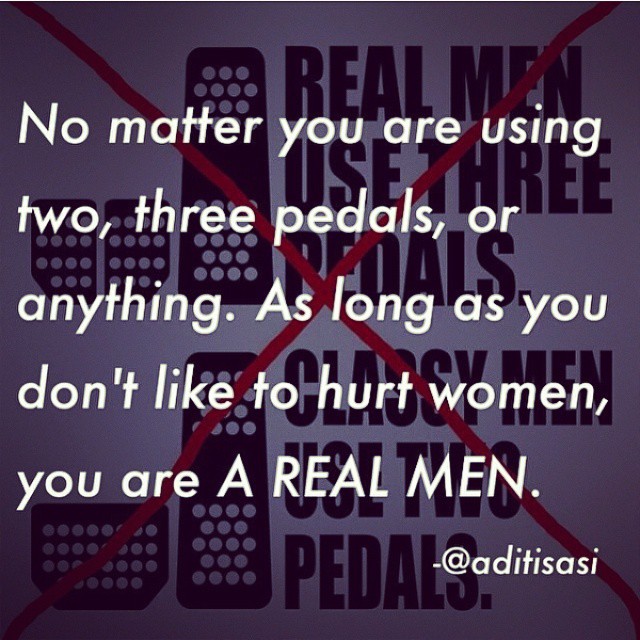This image features a purple background with layered text and graphics. At the top, white letters state: "No matter you are using two, three pedals, or anything, as long as you don't like to hurt women, you are a real man." Beneath this, in black text, it reads: "Real men use three pedals, classy men use two pedals," which is struck through with a large red X. To the left of the black text, there are illustrations of three and two car pedals. The combination of colors purple, dark purple, red, white, and black form a bold contrast, emphasizing the message in what appears to be a social media graphic.